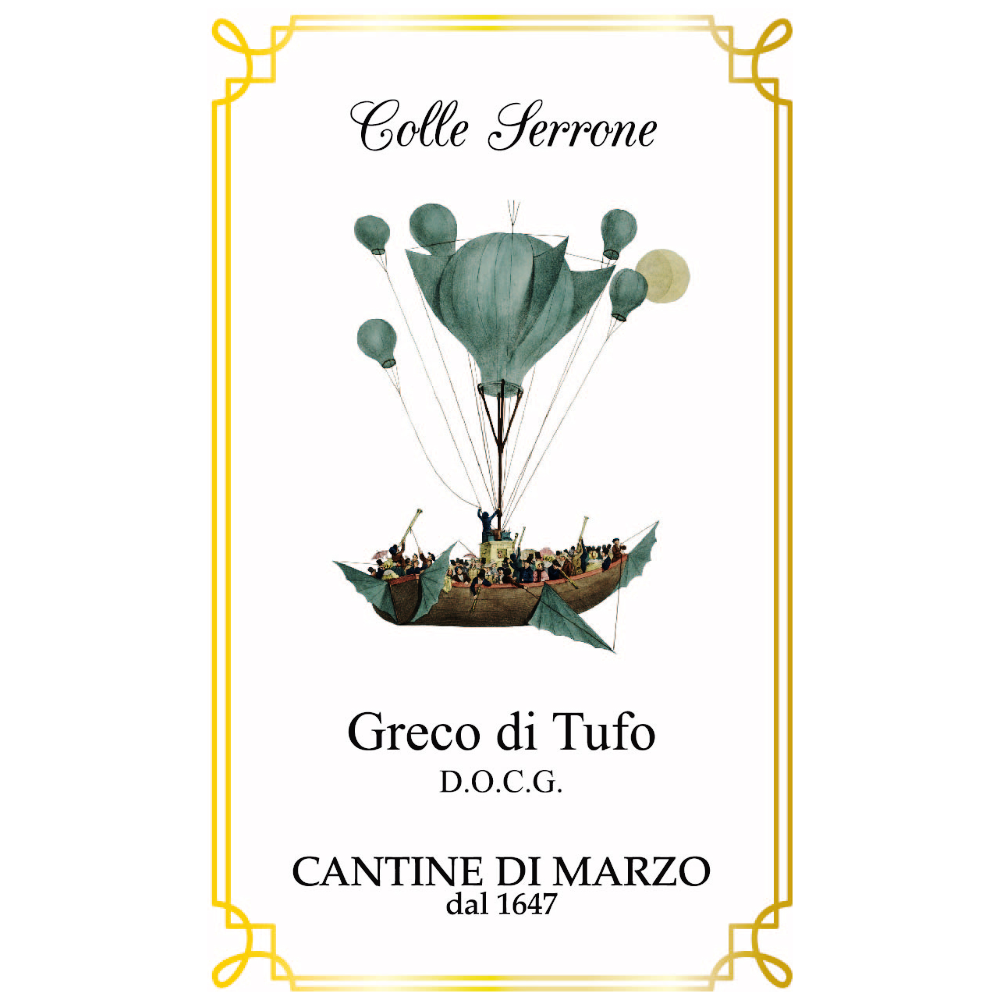The promotional material appears to be an elegant advertisement for "Colle Serrone, Greco di Tufo, D.O.C.G., Cantine di Marzo, DAL 1647." The central image is a fantastical, steampunk-inspired airship fashioned from a large brown rowboat. This boat is adorned with teal-colored wings and is buoyed by a large teal-green hot air balloon with additional smaller balloons. Several individuals are depicted aboard the airship, some holding trumpets or telescopes, fueling a sense of adventure. A creamy full moon forms the backdrop for the airborne vessel. The entire image features a stylish gold double-lined border with intricate loops at each corner. The text "Colle Serrone" appears in a cursive black font at the top, followed by "Greco di Tufo, D.O.C.G.," "Cantine di Marzo," and "DAL 1647" beneath the airship illustration, against a plain white background. The scene exudes a whimsical and vintage atmosphere, perfectly encapsulated within its ornate golden frame.